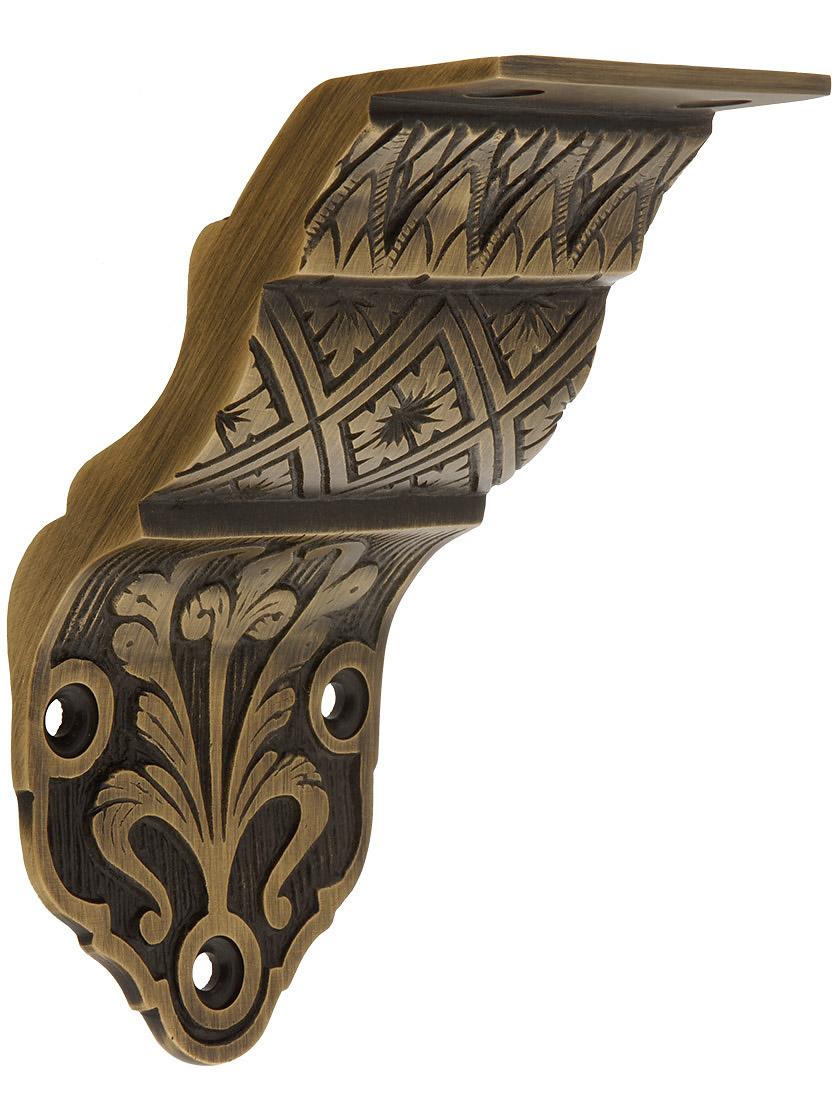The image is of a metal bracket, likely made of bronze or copper, featuring intricate carvings. The metal object, with a brownish hue, is designed to fit in the corner where two walls meet or between a ceiling and a wall. It has a complex, multi-stepped shape: it starts as a vertical bracket, then steps forward and upward multiple times. The lower section has three screw holes, while the upper section has two more, positioned 90 degrees apart to facilitate corner mounting. The piece is elaborately decorated, with the lower part flaunting a fleur-de-lis-like design, and the middle section showcasing a diamond pattern. The top part has a flat, triangular mountain-like design. Presented against a white background, the bracket combines functionality with ornate craftsmanship.